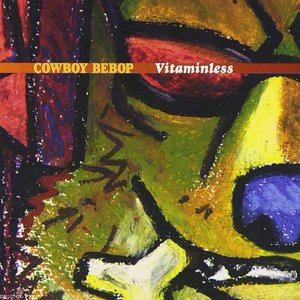The image in question appears to be a vibrant and detailed piece of graphic art, reminiscent of graffiti with bold, bright colors and exaggerated, almost Picasso-like features. The central focus is a close-up of a dog or wolf's face, notably characterized by red eyes and yellow fur. Its mouth partially grins, revealing sharp teeth and a bone. The creature sports a prominent purple nose outlined in dark black and is adorned with black sunglasses that have a red reflection. There is also speculation that the dog might be wearing a motorcycle helmet, suggested by red elements in the upper left-hand corner that could be covering its ears. Spanning across the image is an orange stripe with the words "Cowboy Bebop vitaminless," where "Cowboy Bebop" is written in yellow and "vitaminless" in white, making it resemble an album cover. The overall impression is of a modern, edgy, and vibrant depiction of an animated dog with an attitude, bearing diverse colors and emitting an eclectic, rebellious vibe.